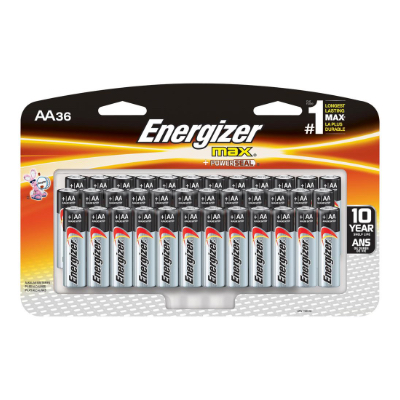This photograph features a pack of AA Energizer Max batteries encased in a notoriously difficult-to-open plastic blister pack. The packaging prominently displays the Energizer branding in the center, accompanied by the Energizer Bunny on the left side. The background is a vivid orange, accentuated by abstract light streaks that resemble lightsabers. In the top left corner, the package is labeled "AA-36," indicating the total number of batteries. Below the Energizer Max logo, descriptive text reads "Power Seal," emphasizing the product's dependable performance. On the right side, a claim of being the "#1 Longest Lasting Max" battery is highlighted, followed by its French translation. The packaging has small triangular holes at the top, designed for hanging on retail racks. Inside, the batteries are arranged in three rows of twelve, organized in this cumbersome blister pack.